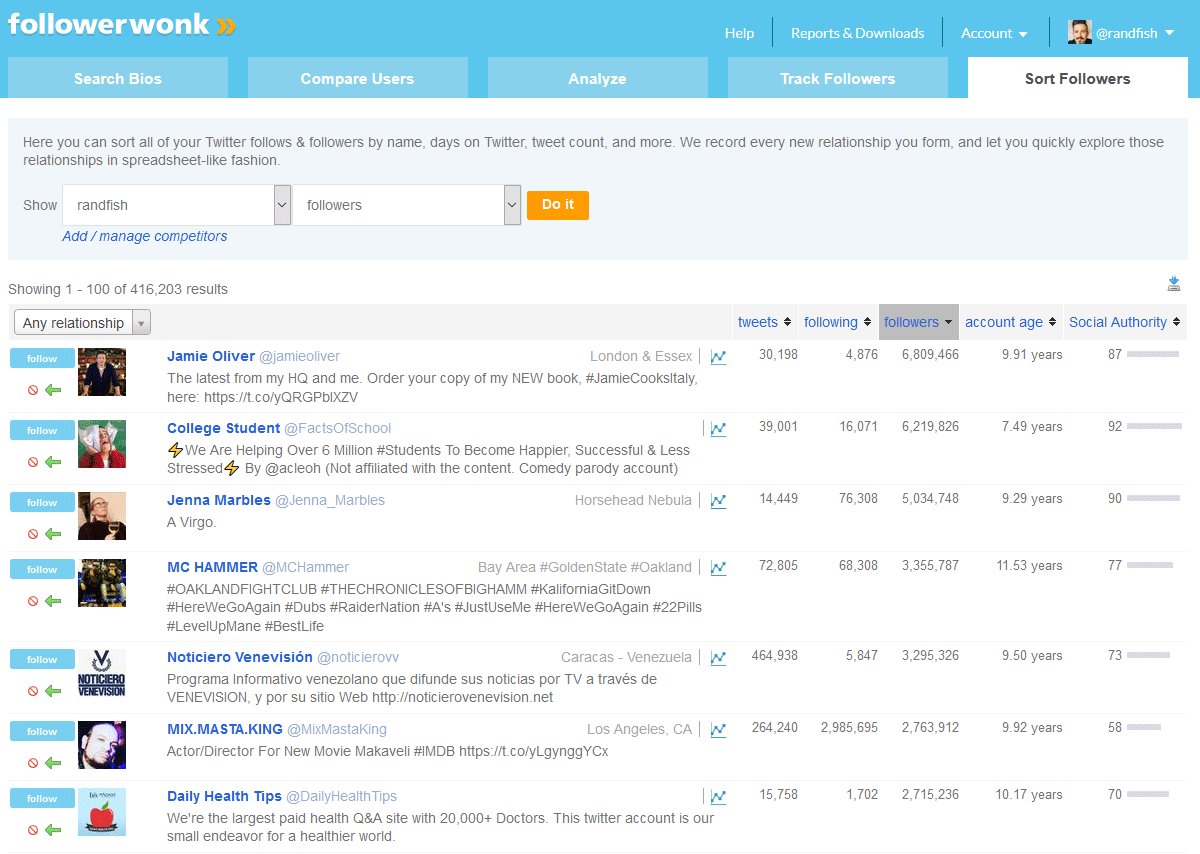This is a screenshot from a web application titled "Followerwonk." The title is displayed in white text in the upper left-hand corner, superimposed on a light blue header banner. The user is logged in as "Rand Fish," whose avatar, a photo of a white man with facial hair, is visible in the upper right-hand corner.

The main section provides a robust interface for managing Twitter followers and follows. It allows users to sort their connections by parameters such as name, days on Twitter, tweet count, and more. Detailed text explains the utility of the tool: "We record every new relationship you form and let you quickly explore those relationships in spreadsheet-like fashion."

Displayed below this informational text is a list of Twitter users following Rand Fish, resembling a spreadsheet. Notable followers include the famous chef Jamie Oliver, YouTuber Jenna Marbles, and musician MC Hammer. This setup underscores the utility of Followerwonk for users managing a significant number of Twitter connections, including high-profile individuals.